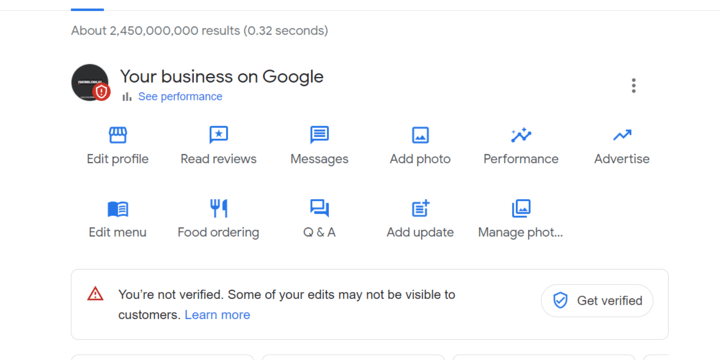This image is a screenshot of a Google My Business web page. At the top of the page, there is a search bar with a blue section on the far left and the rest in gray. The page indicates that there are approximately 2,450,000,000,000 search results. Below the search bar, the headline reads "Your Business on Google" accompanied by an icon which appears either blue or black with white text. Underneath the headline, there is a prominent red circular icon that stands out, and beside it, the text says "See Performance."

There are multiple action buttons listed in blue text, including options such as "Edit Profile," "Read Reviews," "Messages," "Add Photo," "Performance," "Advertise," "Edit Menu," "Food Ordering," "Q&A," and "Update and Manage Photos." These options help users manage their business visibility and engagement on Google.

At the bottom of the page, a large horizontal box spans from the left to the right side of the window. Inside this box is a red triangle with a white exclamation point, indicating a warning message. The message reads "You're not verified. Some of your edits may not be visible to customers." There is an additional note with a "Learn More" link in blue text, which is clickable, and an option to "Get Verified."

On the right-hand side of the page, there is a large circular section, which might be for graphical elements or additional information related to the business profile.